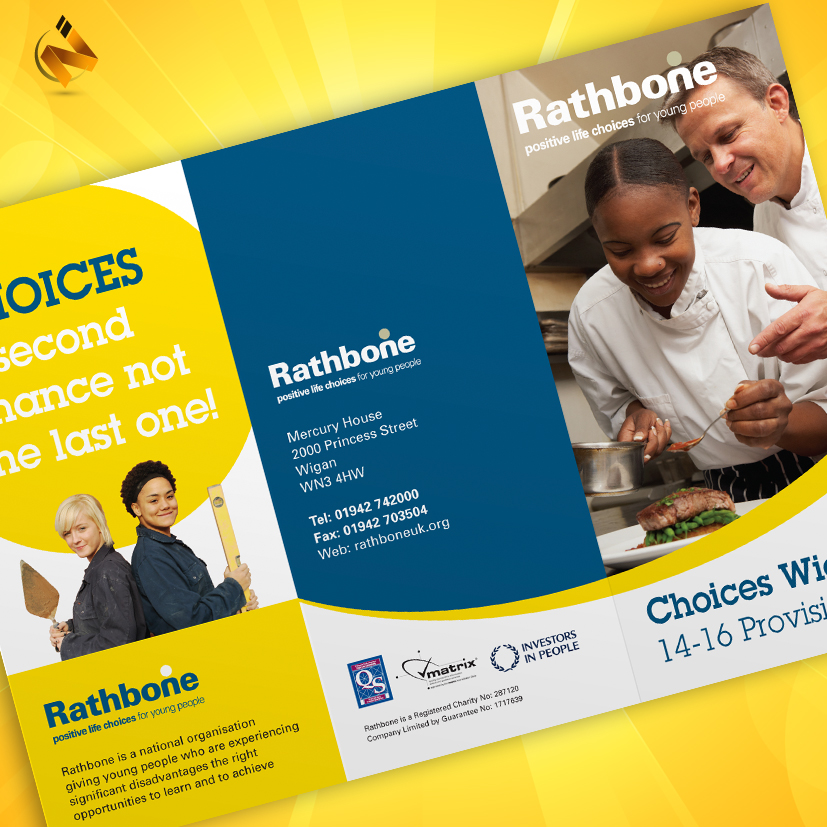The image depicts the front of a Rathbone informational brochure, emphasizing "Positive Life Choices for Young People." Rathbone is a national organization dedicated to providing disadvantaged young people with opportunities to learn and achieve. The brochure is predominantly blue, white, and yellow. At the center, white text on a dark blue background reads "Rathbone Positive Life Choices for Young People," followed by the organization's address (Mercury House, 2000 Princess Street, Wigan WN3 4HW), telephone (0194274200), fax number (01942703504), and website (rathboneuk.org). Rathbone is a registered charity (number 287120) and a company limited by guarantee (number 1717639).

The right side of the brochure features a heartwarming photo of a young black woman in a white chef's outfit, smiling as she pours sauce over a dish, likely steak or salmon. She is guided by an older white man—presumably her instructor—also in a chef’s coat, who gestures encouragingly. Both appear joyful and focused on the culinary task. 

On the left, against a yellow background, two young people are depicted. A young white woman with blonde hair, dressed in a gray coat, holds a spade, while a young black woman with curly black hair, wearing a dark blue coat, holds a level, suggesting engagement in practical vocational activities. This section is accompanied by the text, "Choices: Second chance, not the last one," underscoring the transformative opportunities Rathbone provides. The bottom of the brochure reiterates the organization's mission and contact details, encapsulating its commitment to fostering positive development in young people's lives.